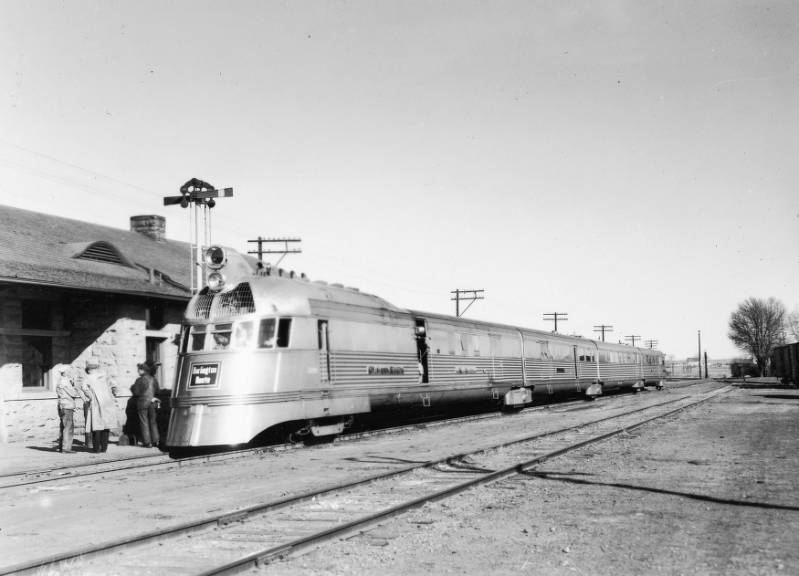This black-and-white photograph, likely from the 1940s, captures a historic, streamlined passenger train at a small outdoor train station. The centrally positioned train, with its engine and several cars, stands on one of the two parallel sets of railroad tracks. To the left of the train is the station building, where a small group of people is engaged in conversation or preparing to board. Above the train, a series of telegraph poles with wires stretch across the scene. In the background to the right, beyond the second set of tracks, lies bare ground, a leafless tree, and another distant building, emphasizing the desolate surroundings. A switching signal is also visible, contributing to the scene's period-specific charm. The photograph captures not only the essence of the train itself but also the minimalistic, utilitarian nature of early 20th-century railway travel.